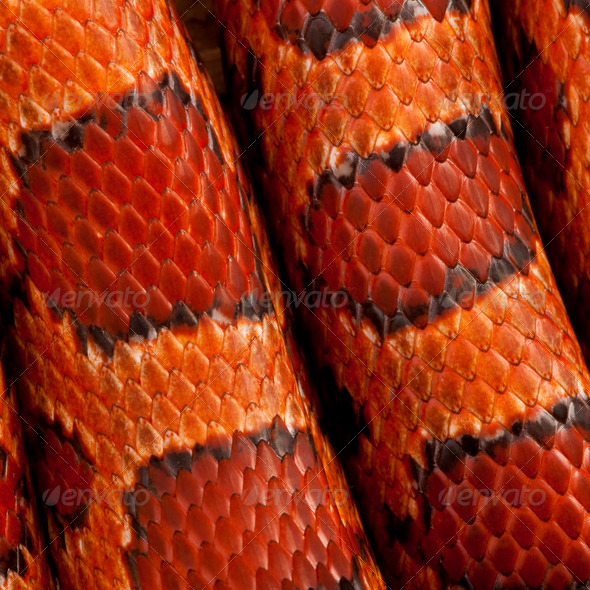This close-up color photograph features a detailed view of the skin of a coiled snake, focusing predominantly on its middle sections. The image showcases the intricate pattern and vivid colors of the snake's scales, which are primarily bright orange adorned with rectangular red spots bordered by black. The dark red to almost black tones further enhance the complex visual mosaic of the snake's skin. These scales, arranged in diamond shapes of a consistent size, appear shiny in places due to the camera flash, highlighting their texture.

The photograph captures multiple segments of the snake's body, suggesting it is either one coiled snake or potentially two resting close together. The heads and tails of the snakes are not visible in this zoomed-in shot. Notably, there are no people present in the image. Watermarks and logos, including the word "Envato" and a water droplet symbol, are lightly scattered in gray text across the image. The settings of the photo are ambiguous but could be either indoors or outdoors, given the focus on the snake's skin.